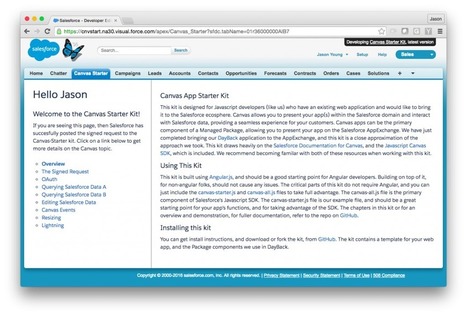This image depicts a screenshot of a browser window with only one tab open. The low resolution makes the URL unreadable, but it seems to be related to "Sky Force" or "Safety Force." The page features a blue cloud icon next to a blue and black butterfly, possibly with the text "Safety Force" written beside it.

Below the main banner, there are several navigation tabs with labels such as Home, Charter, Customs, Campaigns, Leads, Accounts, Contracts, Opportunity Forecasts, Orders, Cases, and Solutions. The currently active tab appears to be "Canvas."

The content of the active Canvas tab greets a user named Jason with the message: "Hello Jason, welcome to the Canvas starter kit." It continues by stating that if Jason is viewing this page, then "Safety Force" has successfully posted a sign request to the Canvas starter kit. The message directs the user to click on a link for more information on Canvas topics, though the exact text is difficult to discern due to poor resolution.